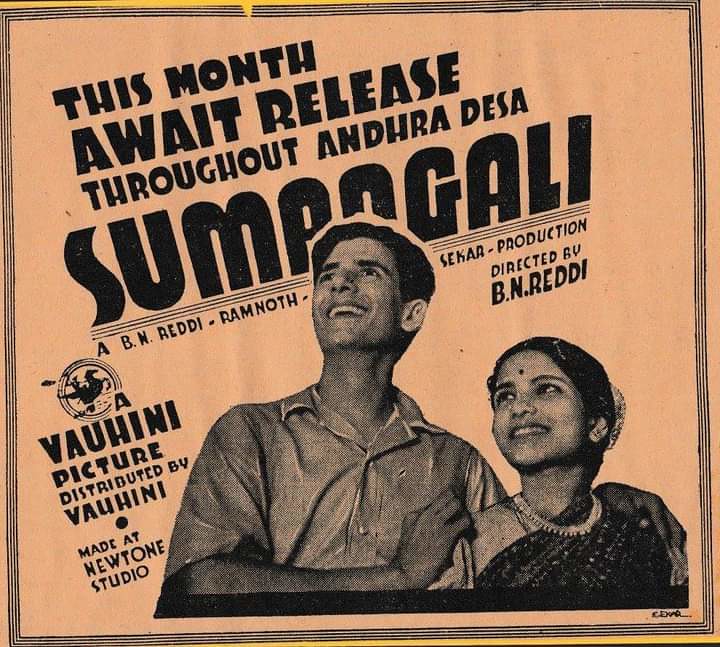The image depicts a vintage movie poster for a Hindi or Bollywood film, possibly from the 1960s or 1970s. The poster is printed in black and white on a peach-colored paper, featuring a distinctive design with three thin black line bars framing the sides. In the bottom right corner, there are images of a man and a woman. The man, with short black hair and wearing a button-up shirt, has his arm around the woman, who is adorned in a traditional Indian dress with a bindi on her forehead. Both individuals are gazing upwards to the left, and the man is smiling.

The background of the poster is plain peach-colored, and the text is arranged in a stylized, sans-serif font with an incline from left to right. The title of the film, "Sumpogali," is prominently displayed, although partially obscured by the man's head. Above their heads, the text reads: "This month awaits release throughout Andhra Desa." Additional information includes: "A BNNReadyRammoth Sakhar production directed by BN Reddy. A Vanuni picture distributed by Vanuni, made at New Tone Studio." A logo featuring a flying horse with a rider is visible on the lower left side of the poster.